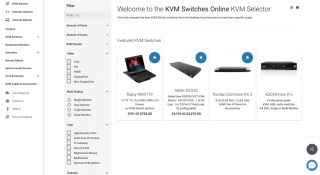The web page features a clean, white background with most of the text in small, unreadable font. At the top, in dark gray text, a prominent header reads, "Welcome to the KVM Switches Online KVM Selector." Directly beneath this header, there is additional text, which is difficult to decipher. Below this text, there is a horizontal row of four images of laptops, each accompanied by a description above and a price listed beneath. To the left of these images, there is a vertical column highlighted in light gray. At the top of this column, the word "Filter" appears in black text, followed by a vertical list of various filtering options with checkboxes. The categories of these options are in bold, but they are too small to read clearly, even when the page is expanded or maximized.